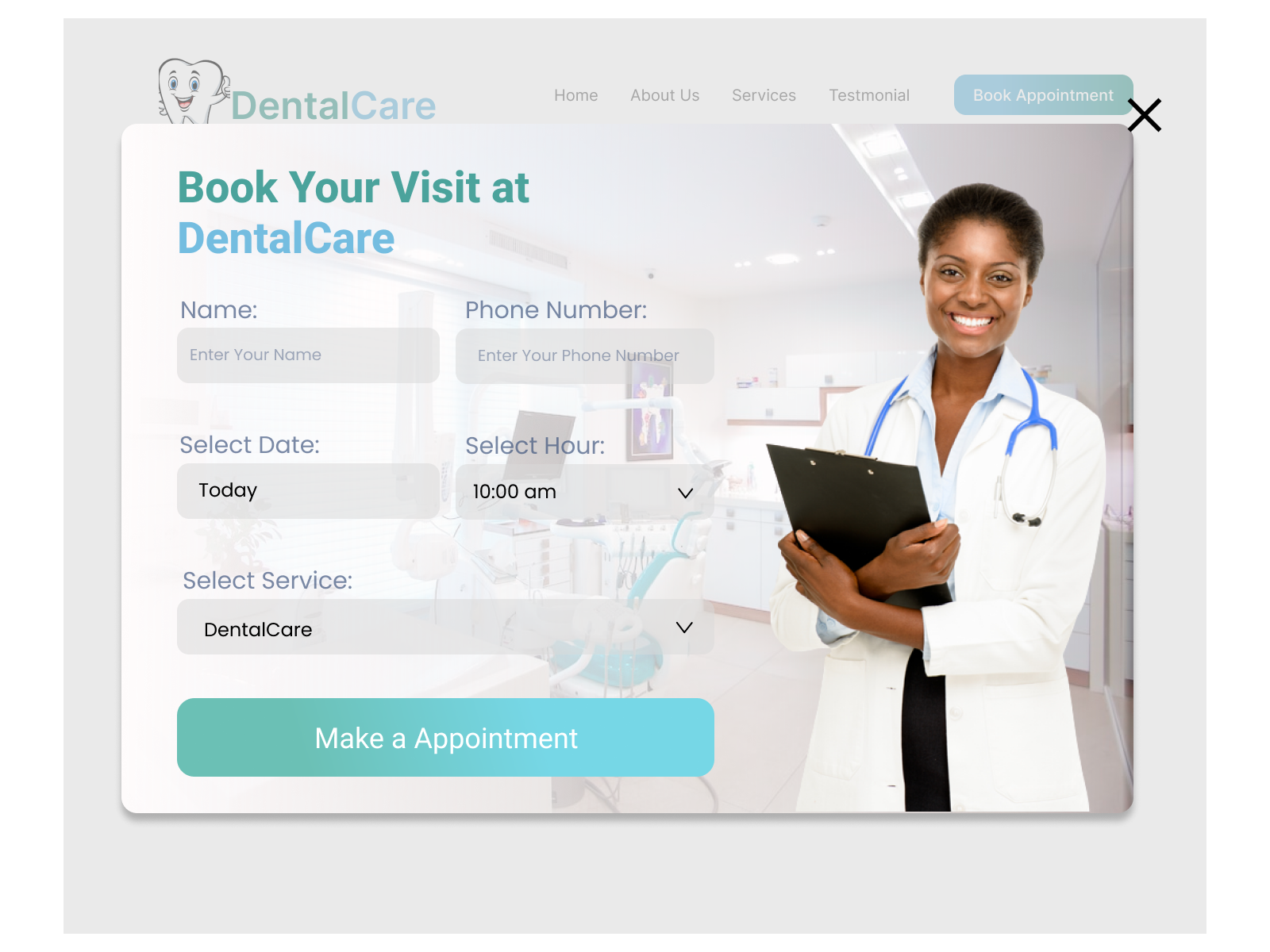The screenshot depicts a booking form on a dental care website. The page features an outer gray background that frames the top, left, right, and bottom edges of the screen. There is no visible URL bar at the top. In the upper left corner, a cartoon tooth with eyes and a smiley face is prominently displayed. To its right, the words "Dental Care" are written in a faint green.

Across the top navigation bar, four labels in black read: Home, About Us, Services, and Testimonial. Positioned on the upper right side is a light blue rectangular button with the text "Book Appointment" in white. Next to this button is a black 'X' symbol, likely for closing a window.

The main content area features an image of a female dentist wearing a white lab coat, holding a clipboard, with a stethoscope around her neck. She is smiling warmly at the camera. To the left of the dentist's image, bolded blue text reads: "Book Your Visit at Dental Care."

Below this heading, the booking form presents familiar fields. The first field labeled "Name" on the top left has a rectangular gray button that prompts users to "Enter your name." Adjacent to it on the right is a field for "Phone Number," also accompanied by a rectangular gray input button.

The subsequent row includes fields to "Select Date" with today's date in bolded black displayed in a gray rectangular button and a dropdown arrow for selecting the hour, which currently shows "10:00 AM" in bolded black.

The final entry field is labeled "Select Service," showing "Dental Care" in a gray background with a dropdown arrow to the right. At the bottom left corner of the page, a long rectangular blue button features the bolded white text "Make an Appointment."